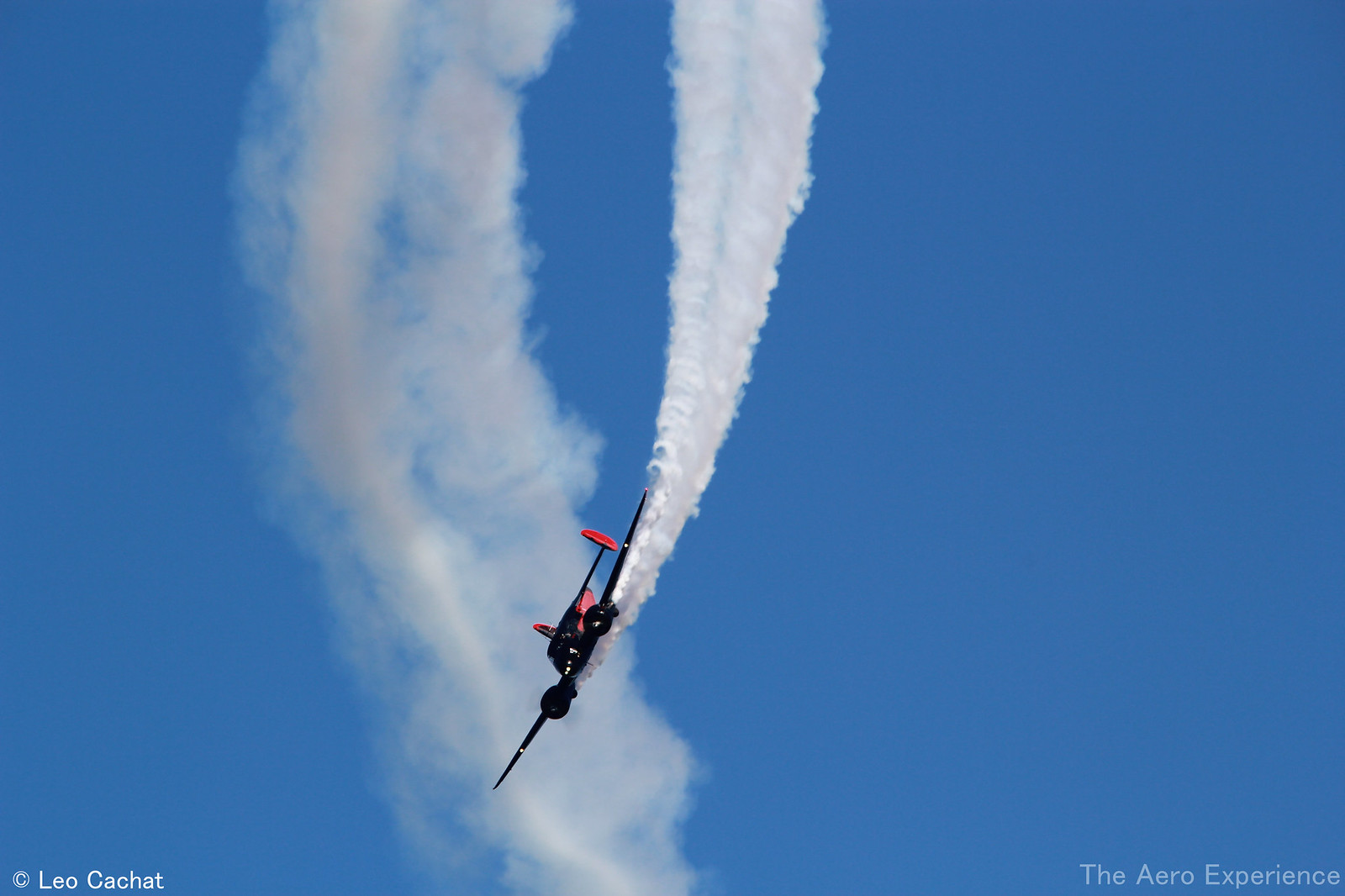This image captures a small reddish-black stunt plane soaring through a crystal blue sky, performing aerial maneuvers with precision and grace. The plane, likely designed for one to two occupants, emits a thick trail of white smoke, curling as if the pilot has just executed a dramatic roll or is in the process of skywriting. In the photograph's bottom corners, there are watermarks: the bottom left reads "Copyright of Les (or Los) Kachat," albeit in small, difficult-to-read white font, while the bottom right bears the mark of "The Aero Experience." The harmonious blend of the vivid blue sky, the dynamic white smoke trails, and the sunlit atmosphere creates an almost postcard-like quality, capturing the exhilarating essence of aerial acrobatics.